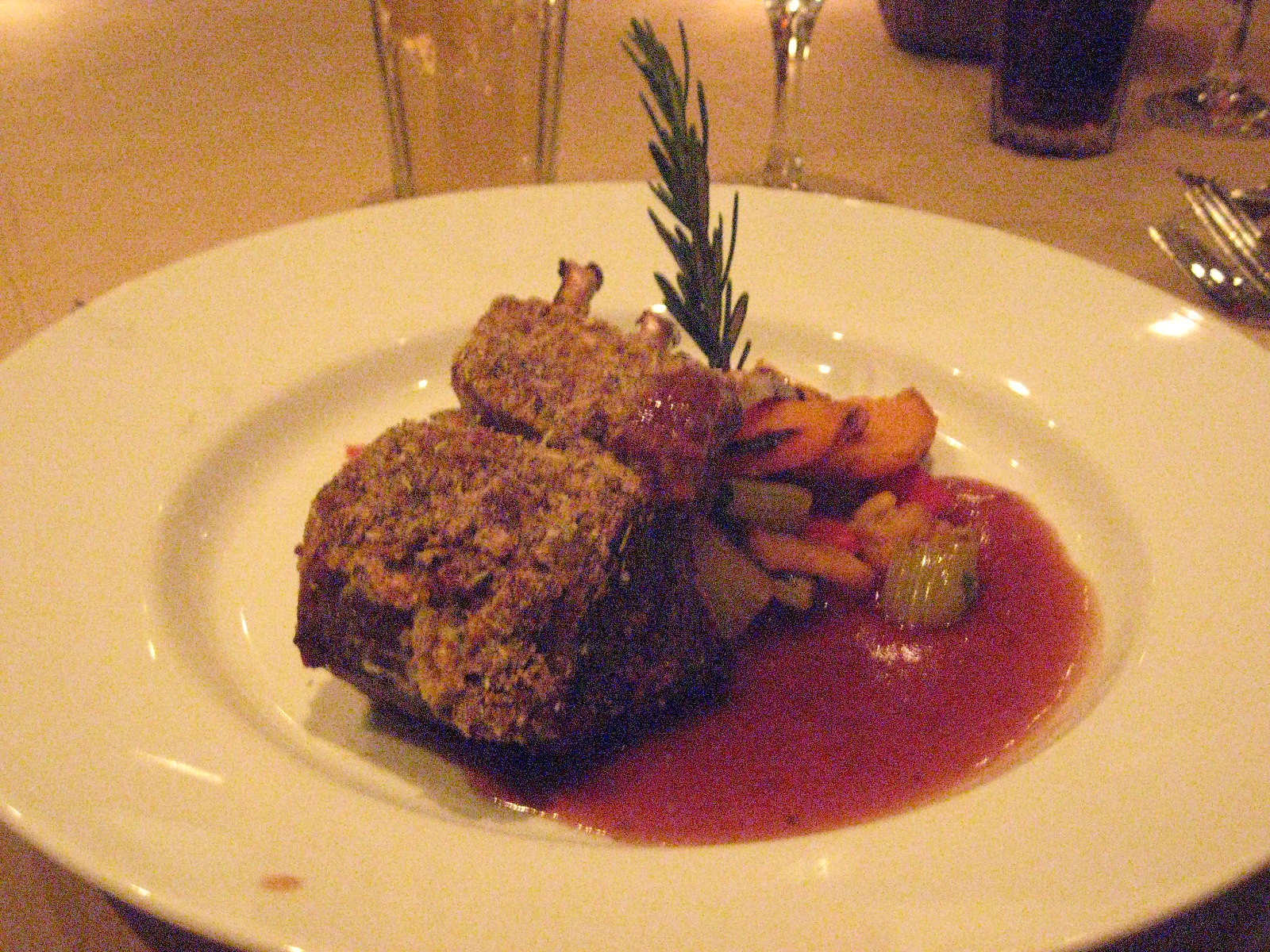This indoor, full-color photograph, taken at a restaurant, features a square composition centered around a white plate of food. The main dish appears to be a piece of beef, crusted with a streusel-like topping and served with a red sauce, possibly jus or gravy. Accompanying the beef are small bits of orange and green vegetables, likely carrots and celery, and a decorative sprig of rosemary. Surrounding the plate are various glasses: in the upper right corner, a glass filled with soda, flanked by what seem to be wine or champagne glasses. Additionally, a clear water glass is visible towards the top left, near a fork and spoon.